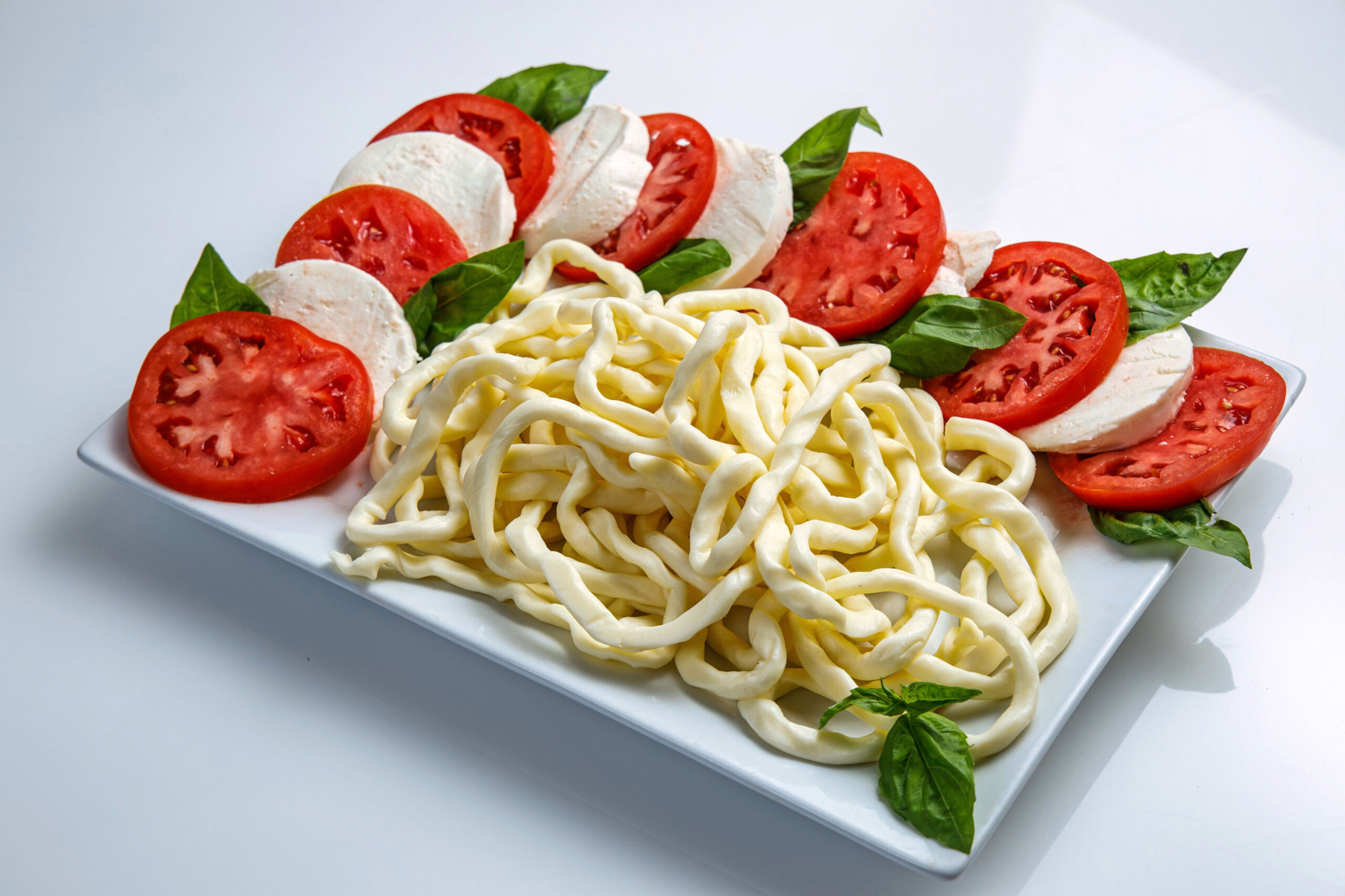The image showcases a slightly indented white rectangular platter on a white countertop, lit from above. Positioned at an angle, the platter prominently features a large clump of white, stringy noodles (or similar food) occupying the bottom right-hand corner. Arranged in an 'L' shape surrounding the noodles are alternating slices of vibrant red tomatoes and white cheese, possibly feta. Interspersed among the tomatoes and cheese are small green leaves, potentially mint or another type of herb, adding a fresh, colorful contrast. The meticulous arrangement of ingredients—a combination of noodles, tomatoes, cheese, and herbs—creates a visually appealing and harmonious presentation.